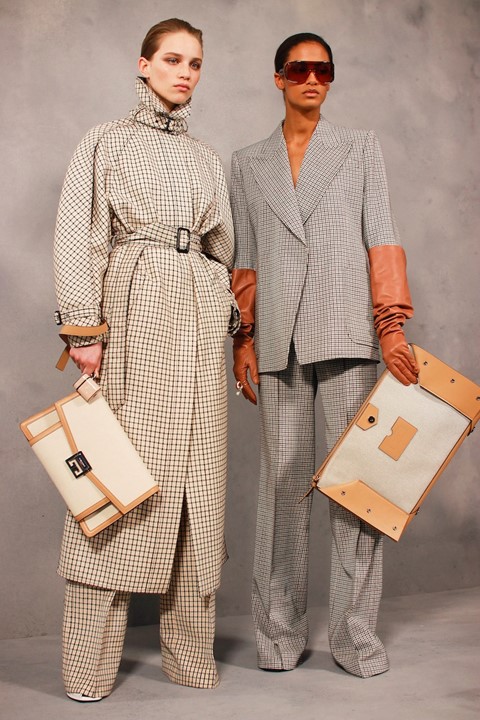This photograph from the Givenchy Fall 2020 collection features two models standing on a gray floor against a gray backdrop. The model on the left, a light-complected Caucasian woman with short brown hair, is attired in a long plaid jacket with matching wide-leg plaid trousers, and barely visible white shoes. She holds a Givenchy purse with a large opening that transitions into a smaller rectangular section, detailed with brown accents and a silver buckle. Her ensemble is cinched at the waist with a plaid belt featuring a dark black brass buckle.

On the right stands a darker-complected African-American woman with short black hair. She is dressed in a gray double-breasted pantsuit, accessorized with long leather gloves that extend to the elbow, one of which sports a ring on the ring finger. She also wears brown sunglasses and carries a larger Givenchy bag, accented with two large brown leather pieces and a central beige element, somewhat resembling a file folder in shape. The coordinated look of both models, accentuated by their sophisticated outfits and luxurious accessories, showcases the timeless elegance of the Givenchy Fall 2020 collection.